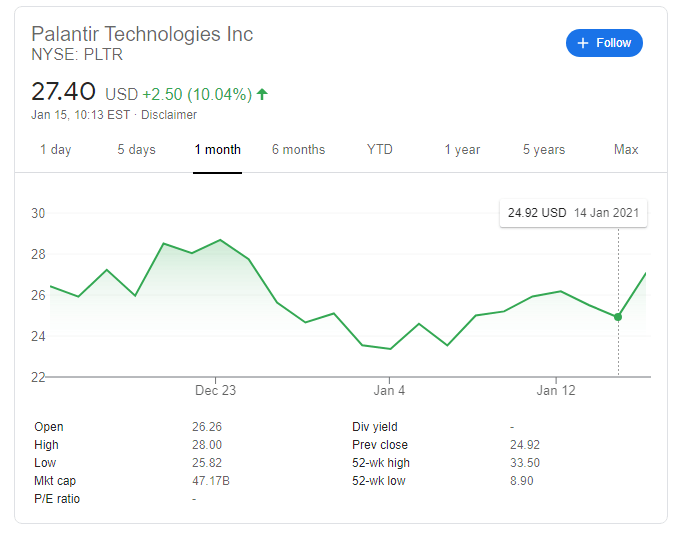The screenshot displays a stock tracker for Palantir Technologies Inc., listed on the NYSE under the ticker PLTR. At the top, the stock price is shown as $27.40 USD. Below, highlighted in green, the tracker indicates a price increase of $2.50, which translates to a 10.04% gain, represented visually by a green up arrow. The timestamp noted is January 15th at 10:13 EST, accompanied by a standard disclaimer. Beneath these details, a green line graph is depicted, illustrating the upward trend of the stock price.